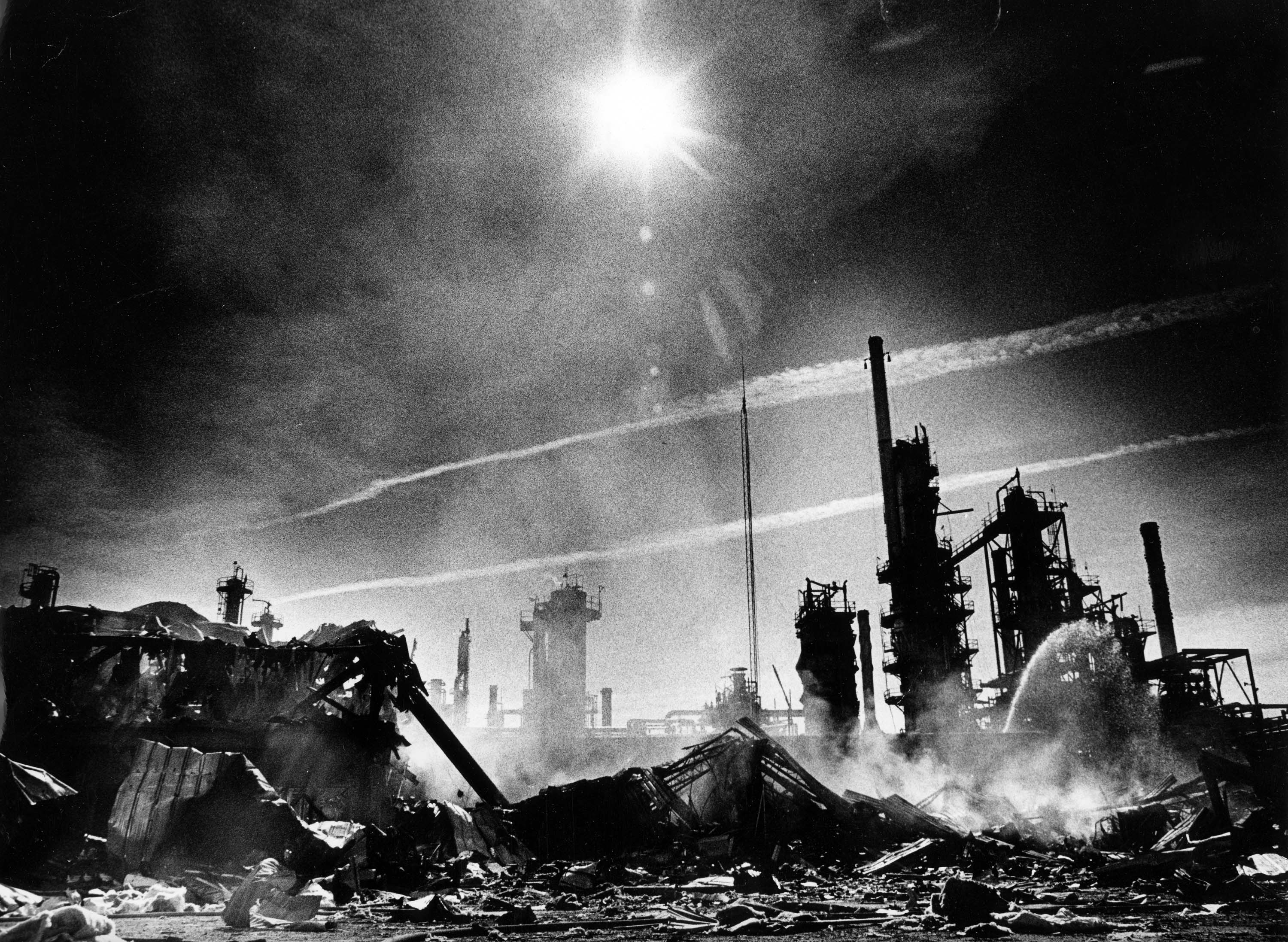This black and white photograph captures a dramatic scene of destruction at an industrial site, likely an oil refinery. The sun, prominently positioned at the top center of the image, casts stark light and shadows across the devastation below. White streaks of clouds decorate the sky, adding to the somber mood. The background showcases intact industrial structures such as cooling towers, flare stacks, and smokestacks, which contrast sharply with the foreground chaos. 

In the foreground, a chaotic pile of mangled metal and rubble dominates the scene, indicating a recent explosion or fire. The remnants of collapsed buildings, including twisted tin sheeting and steel beams, are scattered across the ground. Amidst the rubble, a fire hose sprays water, possibly in efforts to douse lingering flames or cool down smoldering debris. Additionally, a liquid arches up in a spray from the lower right part of the photo, adding to the sense of ongoing emergency response. Smoke or steam rises from the wreckage, further contributing to the dramatic and dire atmosphere of the image.